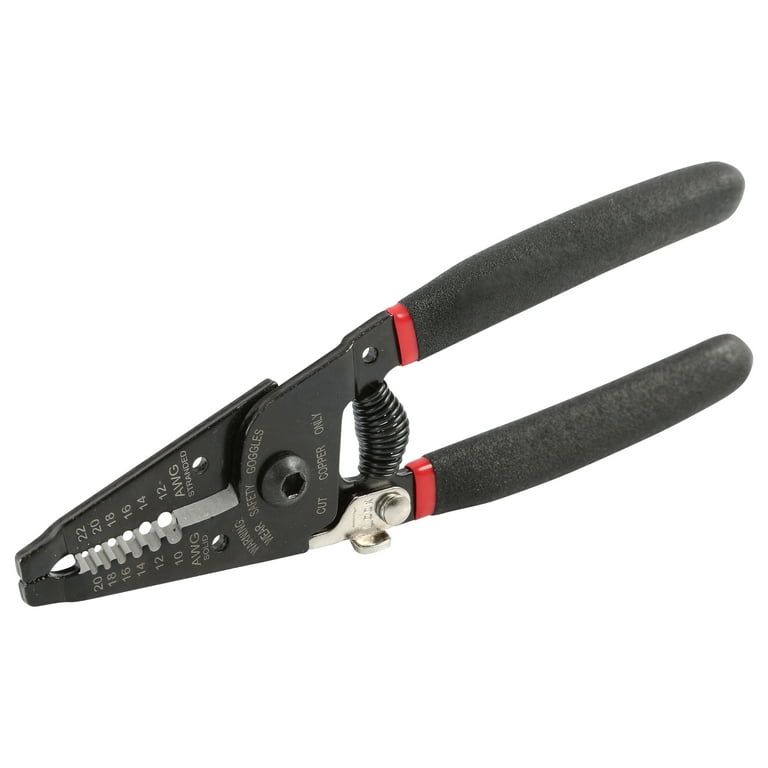This image showcases a high-quality copper wire cutter, prominently featured on a likely e-commerce platform due to the absence of a background. The cutter features a sleek design with a predominantly black body, complemented by soft, ergonomic black handles for comfortable grip. Distinctive red accents are visible near the top of the handles, providing a stark contrast and enhancing its visual appeal. A black spring is positioned between the handles, enabling smooth operation. The cutter's head is adorned with etched numbers indicating wire gauges, capable of handling sizes from 20 to 12 AWG, suitable for both solid and stranded wires. Detailed instructions and safety warnings are inscribed around the central pivot, including "wear safety goggles" and "cut copper only." The tool also features multiple holes for different wire sizes, ensuring precision in usage. The presence of silver elements, including a lever, adds to the instrument's professional look and functionality.